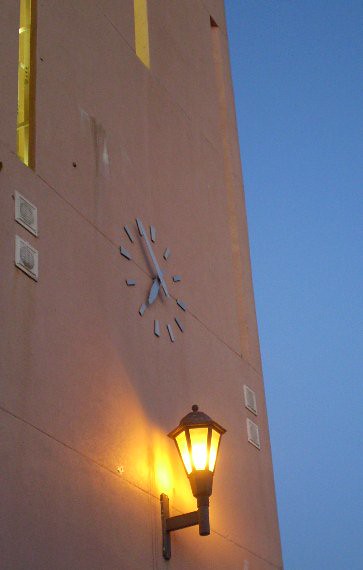This image depicts the upper side of a building, resembling a correctional facility due to its architectural features. The building has tall, narrow windows that suggest a fortified structure. The scene is captured during the evening, as evidenced by the dusky sky visible on the right side of the image. The photograph focuses on the upper section of the building, excluding the roof and the ground. A lantern-style light fixture is affixed to the building, adding a touch of antiquity. Additionally, a clock is prominently displayed on the building's facade, indicating the time as 7:55.